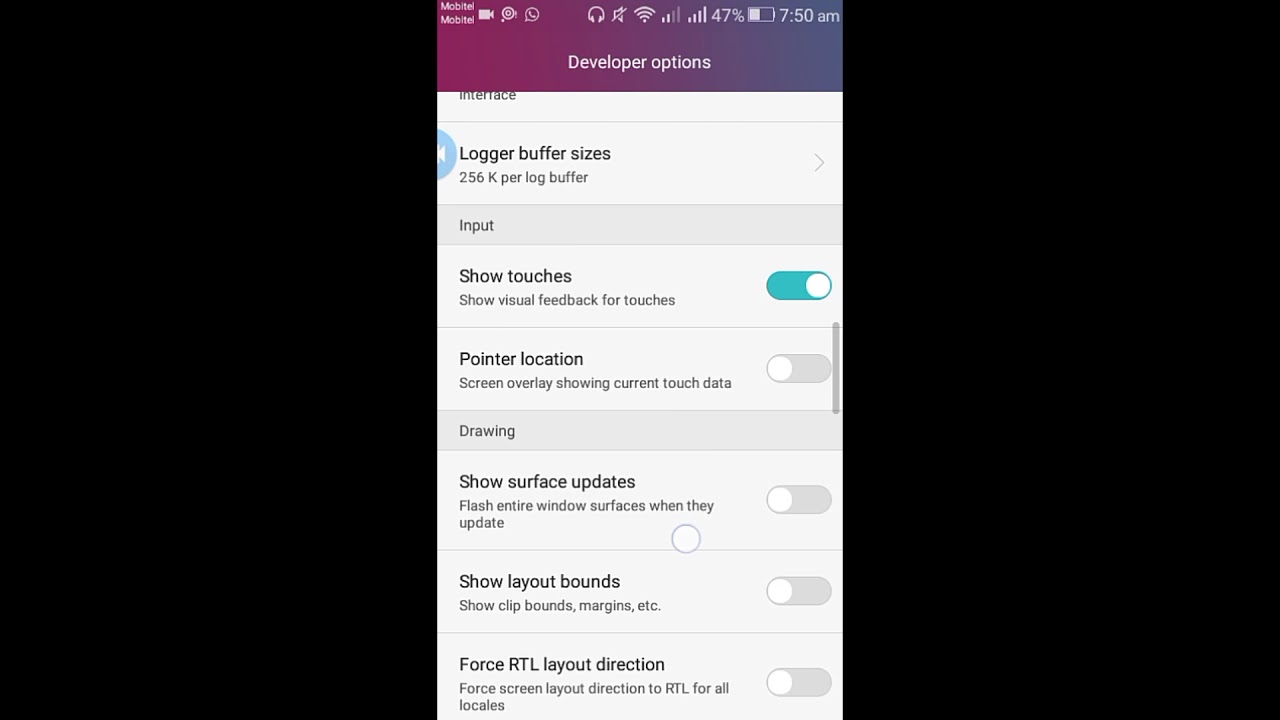The image appears to be a screenshot of a mobile device's developer options menu, displaying several icons and settings. At the top of the screen, there is a headphone icon, a speaker icon with a slash indicating it is muted, a Wi-Fi icon, and a signal indicator showing two out of four bars. The battery level is at 47%, with the device displaying a distance of 750 meters. Developer options are enabled, indicating the device is operating in a specialized mode for testing and debugging.

To the left of the screen, there is a half-circle icon with an arrow, suggesting it can be pulled out for additional options. The menu lists several settings, starting with "Log buffer sizes" set to 256kb per log buffer. Below, a gray bar labeled "Input" includes multiple options:
- "Show touches" toggled on, indicated by a blue oval with a white circle, providing visual feedback for user touches.
- Another setting, "Point of location," displays overlay data for current touch positions, currently not toggled (shown in gray).

Another section labeled "Drawing" includes:
- "Show surface updates" (not toggled), which would flash entire window surfaces when they update.
- "Show layout bounds" and "Show clip bounds" for displaying margins and other layout boundaries (both not toggled).
- "Force RTL layout direction," which forces the screen layout direction to right-to-left for all elements, also not toggled (left side and right side grayed out).

Lastly, there is a microphone icon visible, possibly indicating that voice input is enabled or available.

Overall, the image captures a detailed overview of the developer settings enabled on the mobile device, including various options for logging, input, and drawing validations.